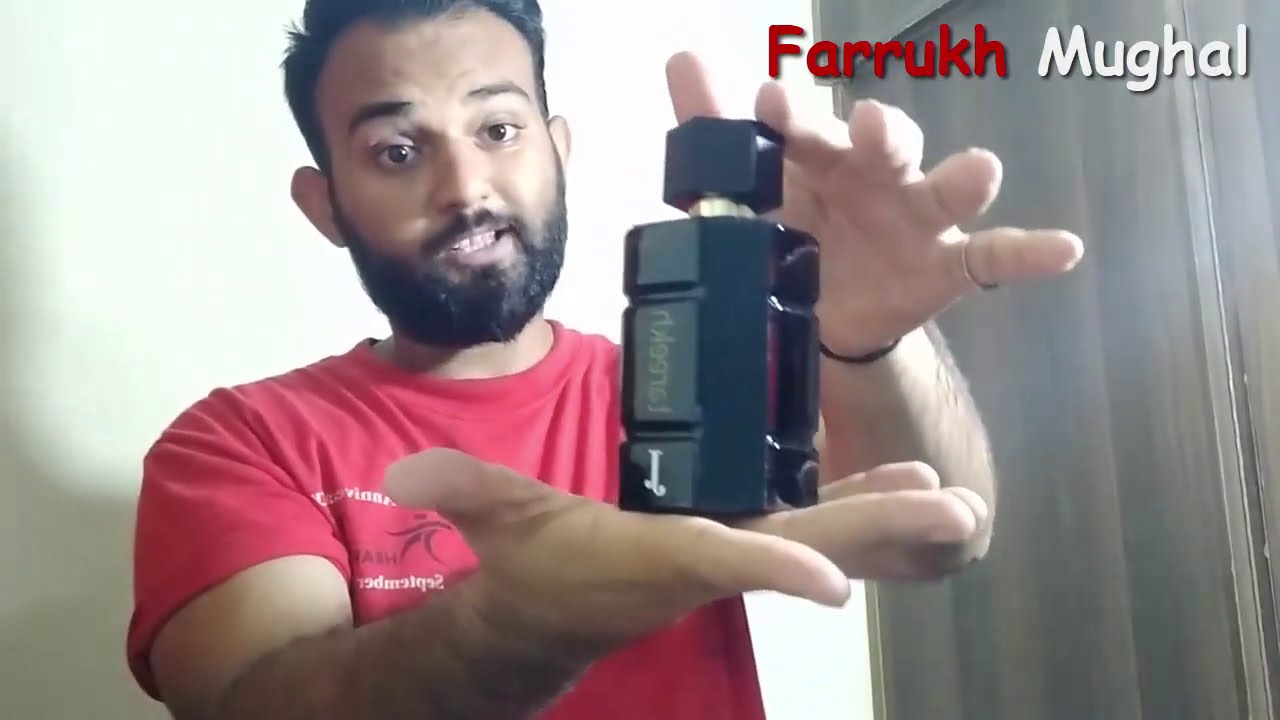In this image, we see a man presenting a small, black, geometric bottle, which appears to be a perfume or cologne, with a black cap and a short gold neck. He holds the bottle in his palm while the other hand touches the cap. The man has short dark hair, a dark beard, and a small mustache, and is wearing a red t-shirt that features a graphic design and some text, though it's difficult to decipher, possibly reading "September". He also wears a pinky ring on the hand touching the cap. The scene is set against a white wall, with a wooden or brown curtain-like object to the side. In the top right corner of the image, the name "Farrukh Mughal" is displayed, with "Farrukh" in red text and "Mughal" in white text. The man is positioned with an open mouth, showing his teeth, and is looking towards the object he is holding.